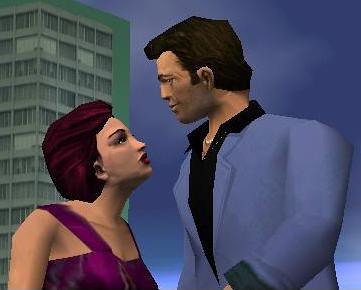In this computer-generated image, a woman is prominently featured on the left side, beginning from the halfway point and extending downward. The viewer sees her right profile, showcasing her short, reddish-purple hair and her vibrant red lipstick. She is clad in a maroon top with thick spaghetti straps. Her gaze is directed upwards towards a man standing to her right. The man, taller than the woman, is observed from his left side. He has dark hair and is dressed in a collared black shirt beneath a gray jacket.

The background behind the woman on the left side of the image reveals a gray building, visible from a corner view, with windows and green accents around the edges. The remaining portion of the backdrop transitions into a serene blue-gray-purple sky, adding depth and contrast to the scene.